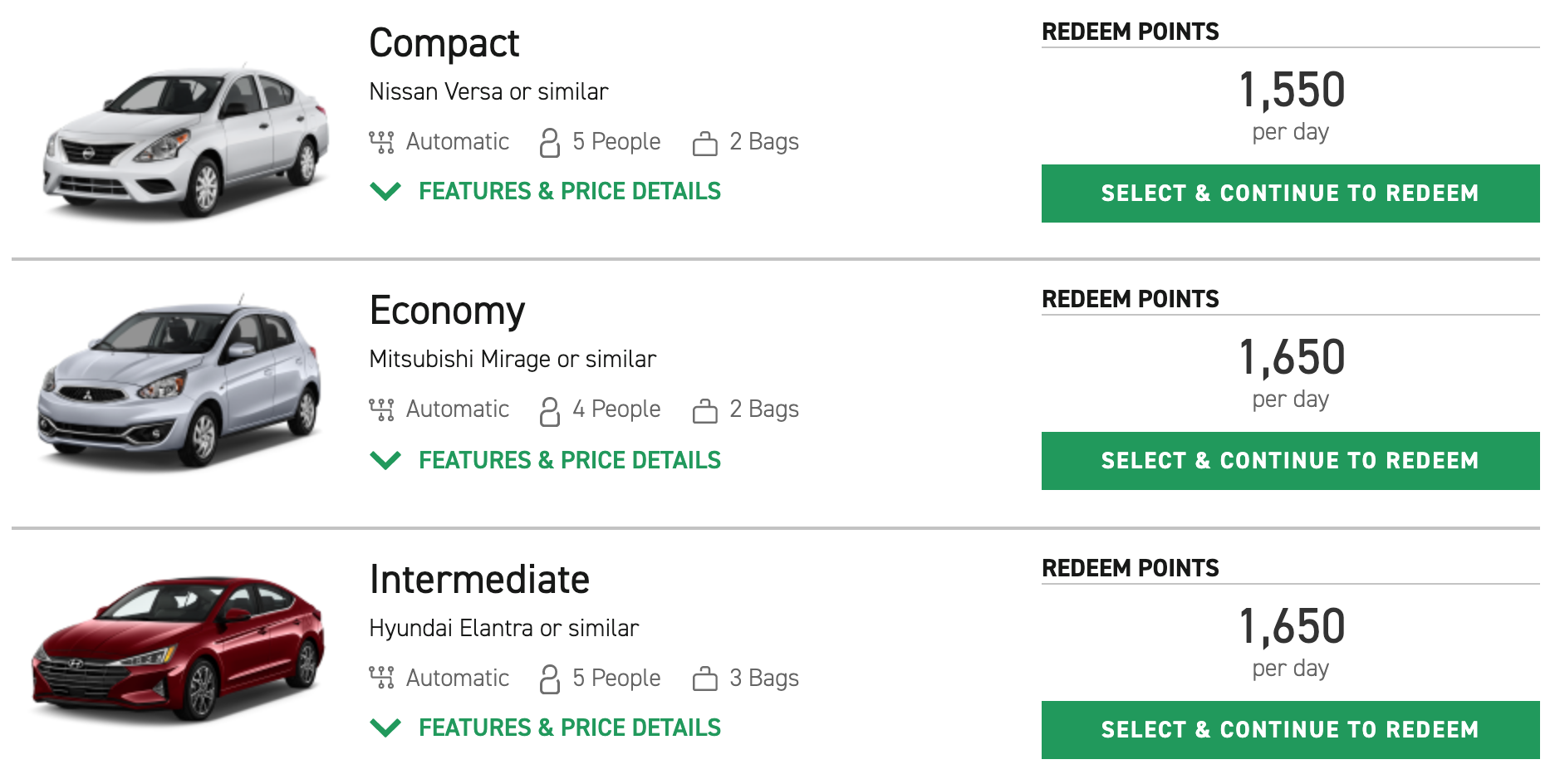The image depicts a car rental website's search results, showcasing various vehicle options sorted by size categories: Compact, Economy, and Intermediate. Each category stacks vertically from top to bottom. 

1. **Compact Car**: 
   - **Model**: White Nissan Versa or similar
   - **Rental Rate**: 1,500 points per day
2. **Economy Car**: 
   - **Model**: Gray Mitsubishi Mirage or similar
   - **Rental Rate**: 1,650 points per day
3. **Intermediate Car**: 
   - **Model**: Red Honda Elantra or similar
   - **Rental Rate**: 1,650 points per day

Each vehicle option is accompanied by an image of the corresponding car model on the left side of the text. In the top right corner of each list item, the rental rate is displayed in terms of redeemable points. Each entry includes a green "Select and Continue to Redeem" button for easy navigation and selection.